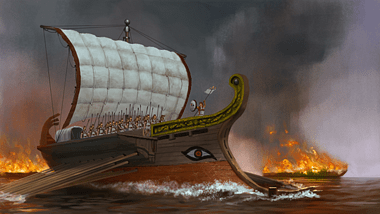This detailed illustration from a book or graphic novel depicts a harrowing scene on the ocean. Dominating the horizontal image is a large, uniquely shaped ship with an eye on its side. The bow curves up and back onto itself, giving the vessel an almost surreal form. A massive sail, detailed with a quilted texture, catches the wind, while several oars dip into the water, propelling the ship forward. Sailors, possibly armed with swords or sharp implements, stand in front of the billowing sail, adding to the tension of the scene. The ship's sides are brown, contrasting with the light and dark grays of the background.

In the distance, two other ships are engulfed in fierce flames, their shapes barely discernible through the thick, dark black smoke that billows into a gradient sky, transitioning from a dark to light gray toward the waterline. The water around the main ship churns, forming white ripples that highlight the motion and urgency as the ship sails towards the right-hand side of the image. The overall atmosphere of the illustration is both intense and grim, underscored by the stark contrast between the burning ships and the muted sky.